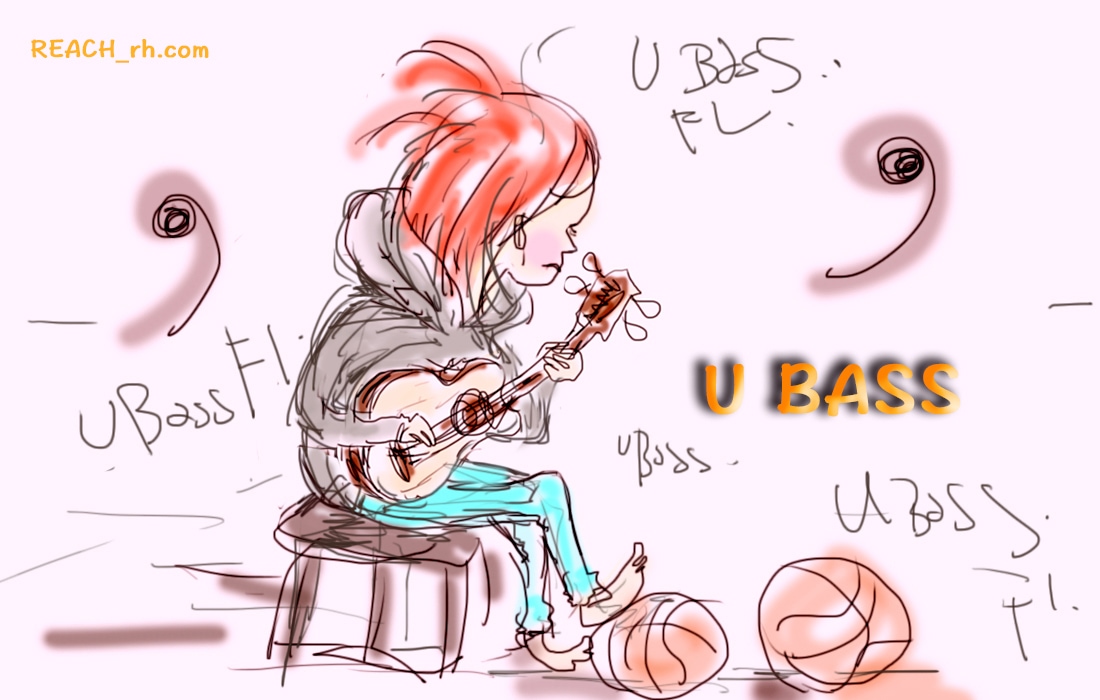The image is a stylized, hand-drawn illustration with a light pink background, featuring a person strumming an acoustic guitar, which has a tan body. The person has long red hair, white skin with a blush, and is wearing a dark gray hoodie and light turquoise (or possibly blue) pants. They are barefoot, with one foot resting on an orange basketball and another basketball nearby. The individual, whose gender is unclear, is sitting on a brown stool and facing to the right, showing a profile view. The art is done with a mix of sketchy ink lines and colorful accents, including some shadowing and shading. Throughout the image, there is text saying "UBASE" in various locations and styles, alongside the text "REACH_RH.COM" in orange in the upper left corner.